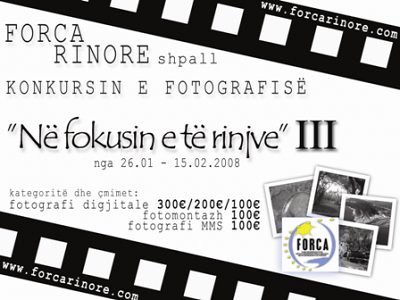The promotional image appears to be for a foreign film or photography event, featuring a detailed and visually engaging layout. The top and bottom edges are designed to mimic old film strips, with black borders and white squares framing the content. These borders feature a recurring website URL www.forcarinore.com. The central part of the image showcases multiple lines of text in a foreign language, possibly a European language. Among the prominent details are mentions of "Forca Inor Sapal Con Cursi e Fotografies" and "Nifoskin et Rimba 3." Additional information includes categories and prizes such as "photography digital: 300€, 200€, 100€," "photo montage: 100€," and "photography MMS: 100€." The bottom-right corner contains small, blurred photographs and a logo related to Forca. Overall, the image serves as an intricate advertisement likely aimed at promoting a photography or film competition.